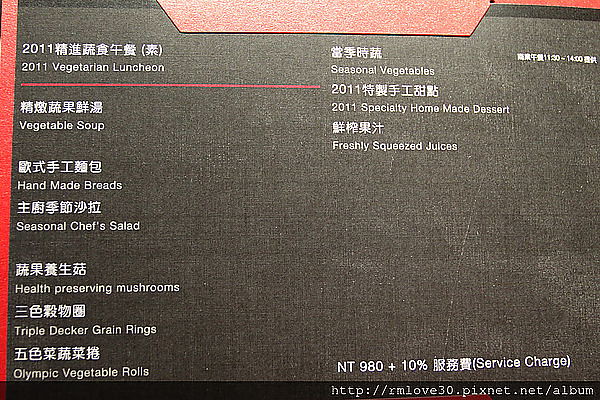The image depicts a rectangular menu card, approximately four inches wide and three inches high, with a distinct black cardstock featuring a paper texture. The card is bordered by a red painted wall, which includes a thin red vertical stripe on the left-hand side and a red parallelogram extending from the top center towards the right. The menu itself is presented in both an Asian language (likely Chinese) and English, with each dish name preceded by its Asian counterpart.

At the upper left corner, the card reads "2011," followed by "2011 Vegetarian Luncheon." Below this, a thin red pinstripe runs horizontally across the card. The menu entries, listed from top to bottom, include: 

1. Vegetable Soup
2. Handmade Bread
3. Seasonal Chef Salad
4. Health-Preserving Mushrooms
5. Triple Decker Grain Rings
6. Olympic Vegetable Rolls
7. Seasonal Vegetables
8. 2011 Specialty Homemade Dessert
9. Freshly Squeezed Juices

At the bottom of the card, it states the price: "NT 980 plus 10% service charge." Additionally, a web address is provided in white print on a thin black footer at the bottom: "http://rmlove30.pixnet.net/album."